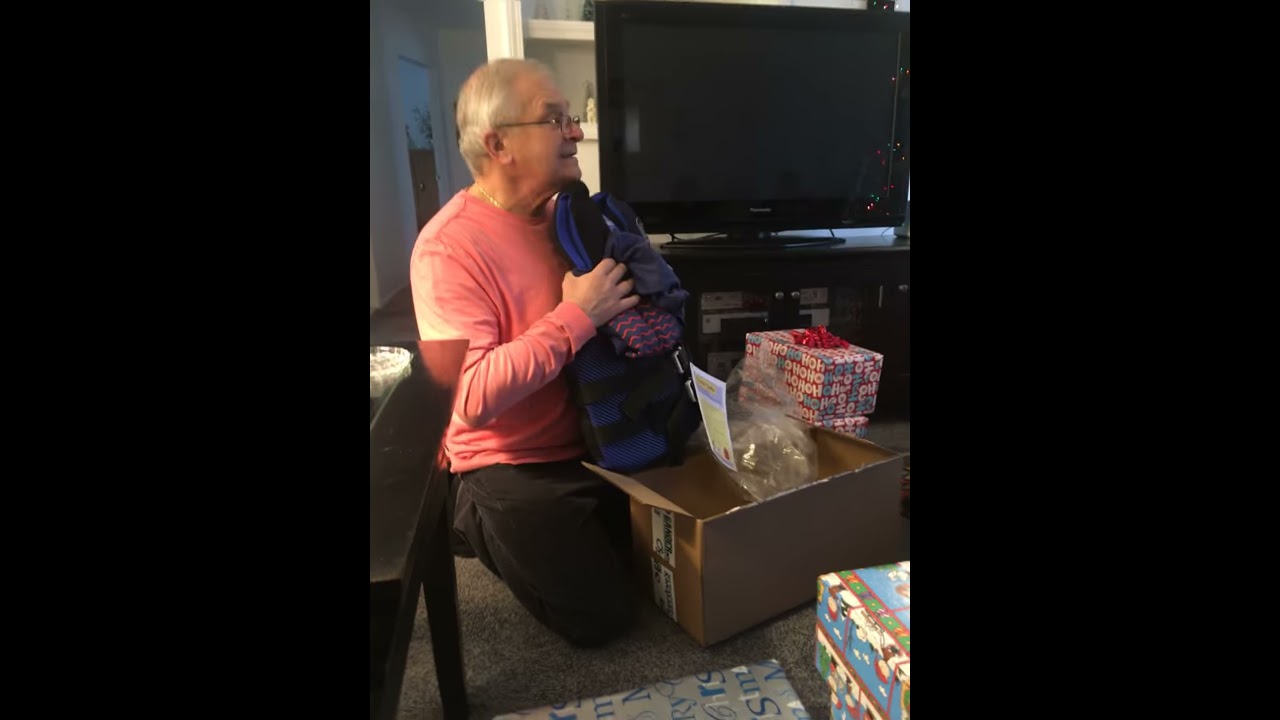In this indoor photograph, an elderly man with white hair and glasses is seen kneeling on the carpeted floor, facing slightly to the right. He is dressed in a pink long-sleeved t-shirt and black pants. The man holds a blue and black backpack in one hand and another blue item, possibly a life jacket or clothing, in the other hand. In front of him lies an open cardboard box with some plastic packaging. Surrounding him are various Christmas presents, including one prominently wrapped in red, blue, and white paper that says "Ho Ho Ho" with a red bow. Behind him, positioned on a wooden table, is a large black flat-screen TV, and nearby are white shelves. The setting of the scene appears to be a dimly lit residential living or family room. The man has a slight smile on his face, adding to the warmth of the scene.